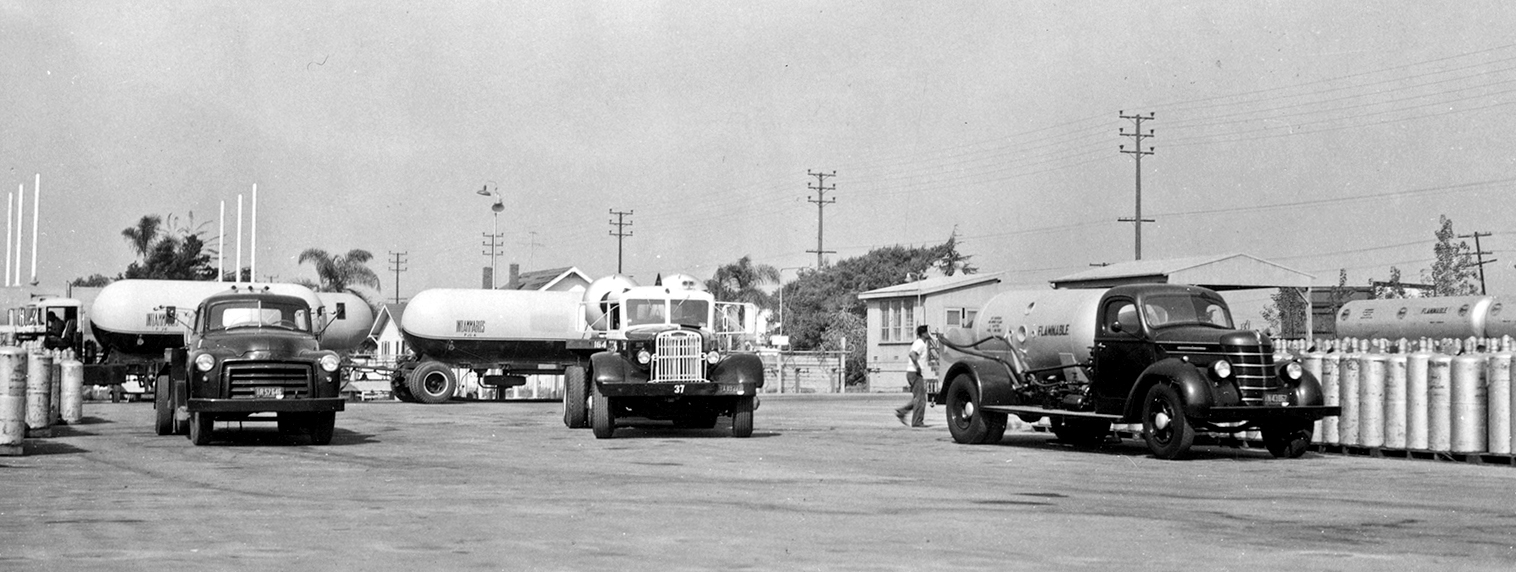This panoramic black and white photograph captures a vintage truck stop scene from the 1950s or 60s, evident from the bubbly, old-school design of the vehicles. The image showcases a flat expanse with multiple trucks, all of which have long cylindrical tanks in the back – these tanks vary in color, with the prominent one on the right labeled 'flammable.' The truck positioned centrally has a distinctive white top and black bottom. To the left, another truck is visible with two such tanks, while several cylindrical canisters cluster on both sides of the trucks. In the far horizon, telephone poles with connecting electrical wires stand tall, and trees and houses form the background. Amid this industrial yet tranquil setting, a lone person in a white top and dark pants walks behind the rightmost truck, adding a human element to this otherwise mechanical tableau.